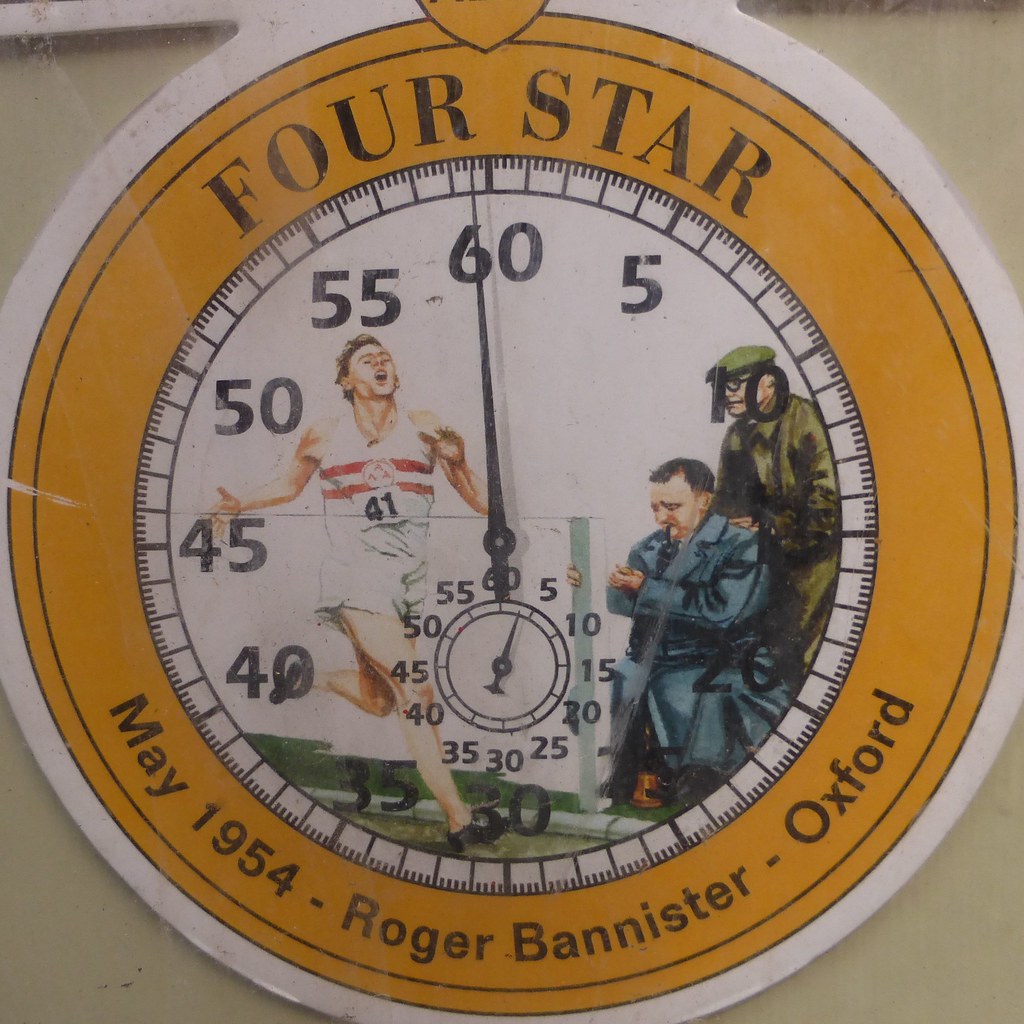The image showcases an old, hand-painted stopwatch encased in an aged, possibly dirty piece of glass. The circular stopwatch is bordered in white and yellow, featuring the text "Four Star" at the top and "May 1954, Roger Bannister, Oxford" at the bottom. The central image depicts a historical moment: a young man, wearing a white sleeveless shirt with two red stripes and the number 41, appears to be finishing a race, with his arms stretched back as he crosses the finish line. To his right, a man in a blue overcoat sits, seeming to time the race with a watch in hand, while another man, dressed in green, stands behind him. The stopwatch includes two smaller dials, one for minutes and one for seconds, with the primary hand halted near the 60 at the top of the clock face. The outer dial counts in increments of 5, from 30 at the bottom to 60 at the top, both clockwise and counterclockwise. The detailed portrayal evokes the era of the 1940s to 1960s.